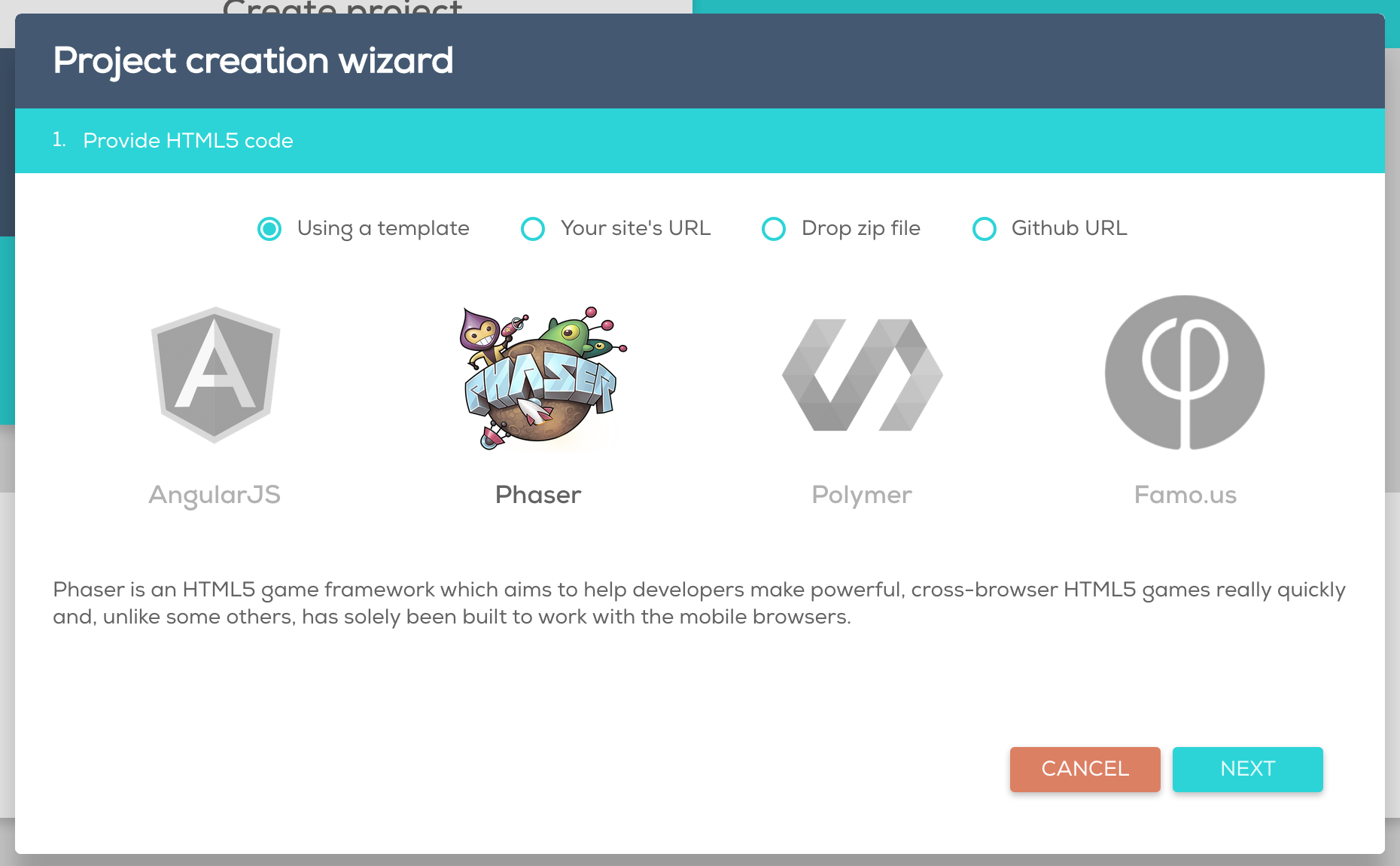The image is a screenshot from a game development software interface. At the top of the image, there are multiple overlay screens. 

The furthest screen in the background displays a simple interface with the text "Create Project." 

Overlaying this background screen is another window with a gray title bar labeled "Project Creation Wizard." Below the title bar is a blue horizontal rectangle that stretches across the screen. Written in white text within this rectangle is step one of the setup process: "Provide HTML5 Code."

Beneath this, there are four horizontal options for the user to select a method to provide the HTML5 code: 
1. Using a Template
2. Your Site's URL
3. Drop Zip File
4. GitHub URL

Each option has a clickable circle next to it, allowing the user to select their preferred method.

Further down, there are various logo options for different frameworks or libraries, displayed horizontally. These include:
- AngularJS
- Phaser
- Polymer
- Famo.us

The Phaser option is currently highlighted. Its logo features a planet with the text "P-H-A-Z-E-R" written above it, surrounded by animated character elements.

Overall, the image shows a structured user interface for initiating a new project in a game development environment, providing various options for code input and framework selection.